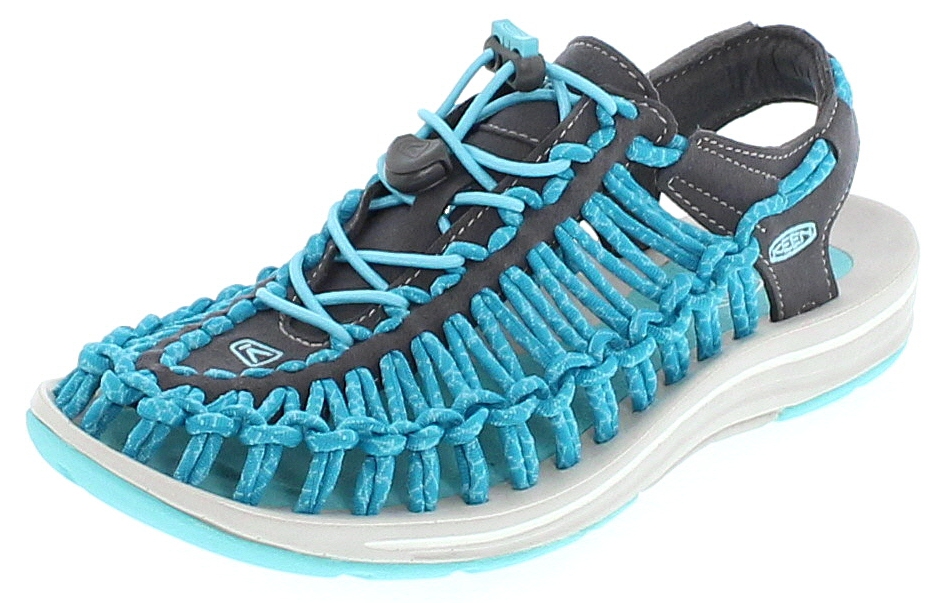This detailed photo captures a unique, sandal-like shoe designed for breathability and versatility, perfect for summer or beach outings. The shoe features a striking combination of colors and materials: the sole is predominantly white with a hint of light blue trim around the heel, while the main body of the shoe is black. Aqua-colored ropes intricately lace through the sides of the sandal, threading from the top and creating symmetrical knots that secure pairs of ropes at regular intervals. These laces, resembling shoelaces, crisscross over the top, suggesting an adjustable size for a customized fit. The shoe also displays a subtle 'K' monogram, adding a touch of branding, and is positioned in a sideways-facing-left orientation, highlighting its detailed craftsmanship and thoughtful design.